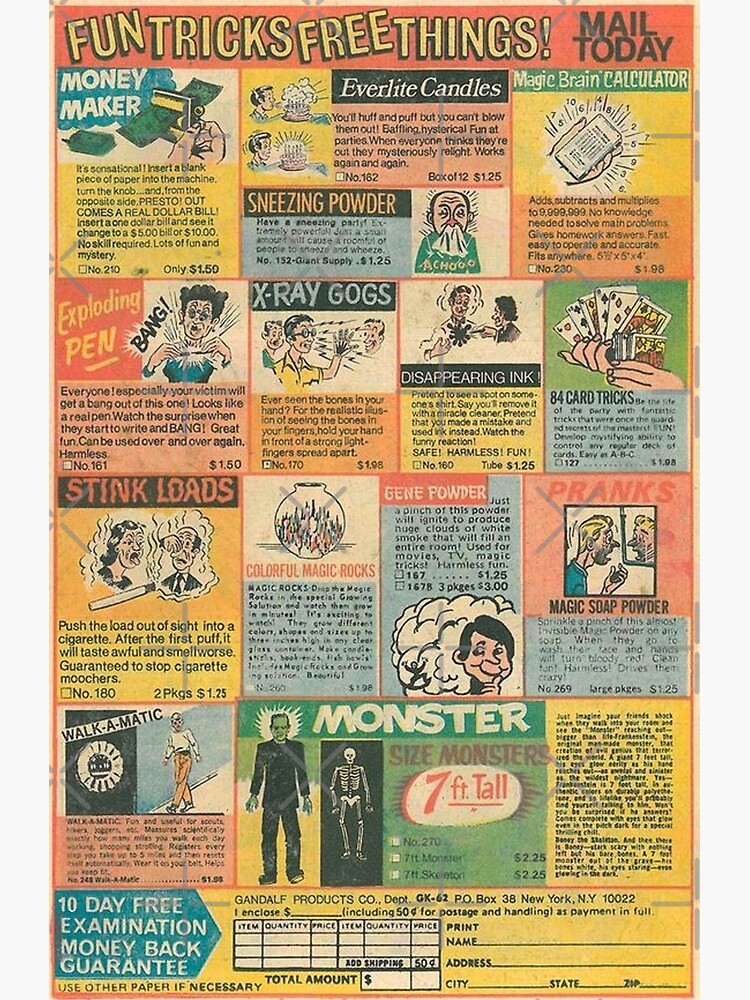This colorful advertisement, reminiscent of the back cover of an old newspaper or comic book, invites readers to mail in a small fee for an array of whimsical and prank items. Dominated by muted yet vibrant shades of yellow, pink, orange, blue, green, and red, the advertisement teems with playful and nostalgic charm. At the top, bold letters announce “Fun, Tricks, Free Things, Mail Today.” The page showcases an eclectic mix of novelty items and practical jokes: a money maker, Everlight candles, a magic brain calculator, sneezing powder, an exploding pen, x-ray goggles, colorful magic rocks, and even stinky loads for mischievous pranks. Items are affordably priced around $1 to $2, hinting at the advertisement's vintage nature. Among the standout offers is a towering seven-foot monster, likely a toy, and a promise of a 10-day free examination with a money-back guarantee, making this a treasure trove of silly, entertaining products appealing to children and collectors alike.